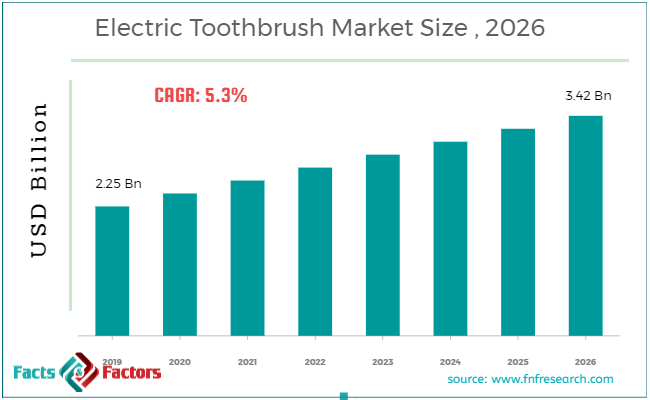The image features a detailed bar graph titled "Electric Toothbrush Market Size, 2026" produced by Facts and Factors Research. Displayed against a white background with simple text, the graph documents the electric toothbrush market's growth trajectory from 2019 to 2026. The vertical axis is labeled "USD Billion" and measures the market size in billions of dollars, while the horizontal axis marks the years: 2019 through 2026. Each year is represented by a teal-colored bar, showing a steadily increasing trend from an initial value of 2.25 billion in 2019 to a projected 3.42 billion by 2026. The graph highlights a Compound Annual Growth Rate (CAGR) of 5.3%, prominently indicated in bold red font. In the bottom-right corner, the source is cited as "www.fnfresearch.com" in blue lowercase font, accompanying the Facts and Factors brand logo with a yin-yang-inspired symbol. This comprehensive graph illustrates the consistent growth and promising future of the electric toothbrush market over the analyzed period.